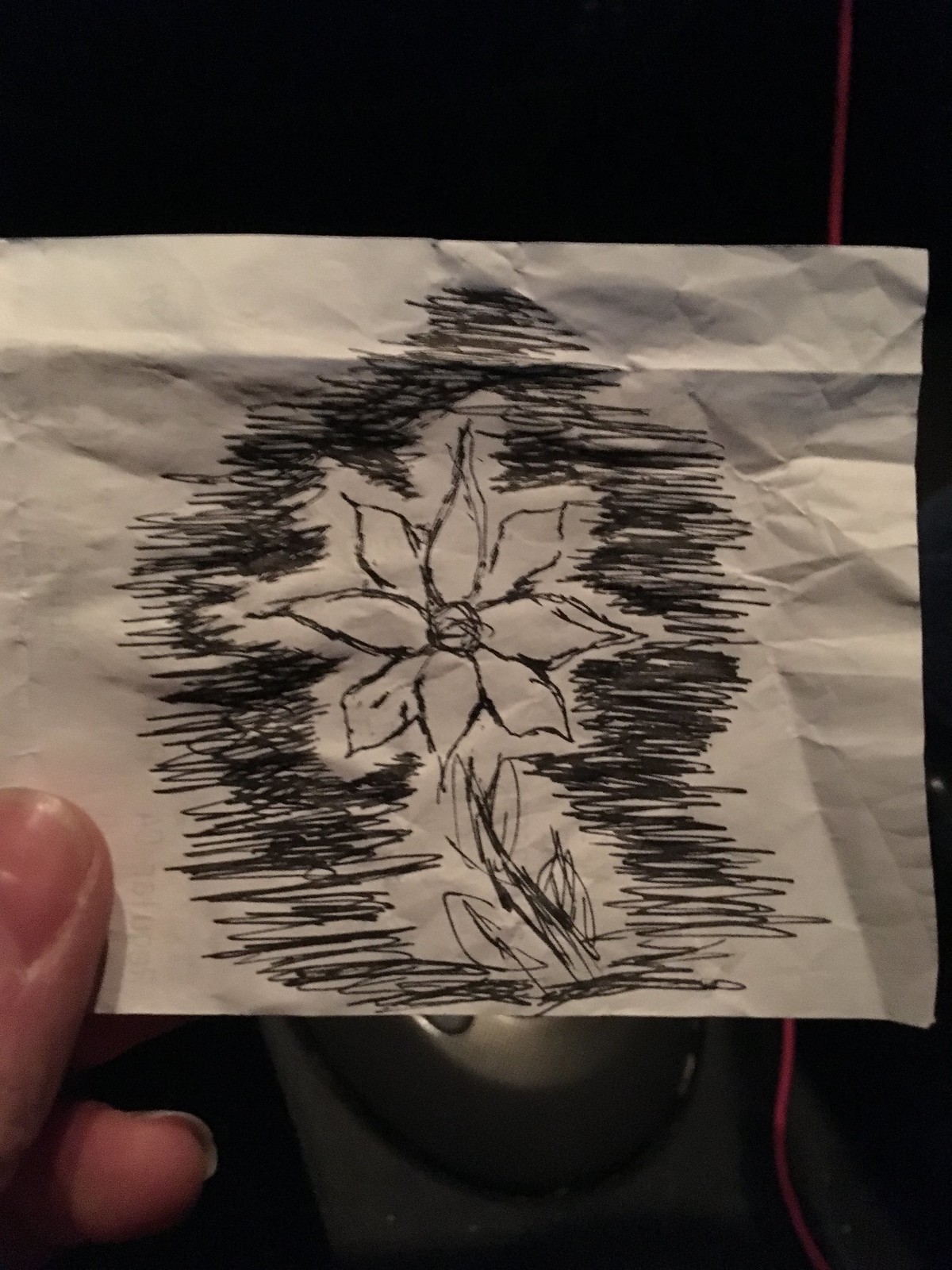In this dimly lit photograph, the focal point is a badly crumpled white receipt being held up by a Caucasian person's thumb and index finger. The receipt, viewed from the back, reveals faint and partially obscured printing typical of store transactions. Amid the wrinkles and creases, there is a poorly drawn illustration made with black ink. This impromptu artwork consists of messy scribbles, with a rudimentary flower in the center. The flower includes basic petals and a chaotic scribble intended to represent the stem, adding a peculiar, almost child-like touch to the otherwise mundane piece of paper.